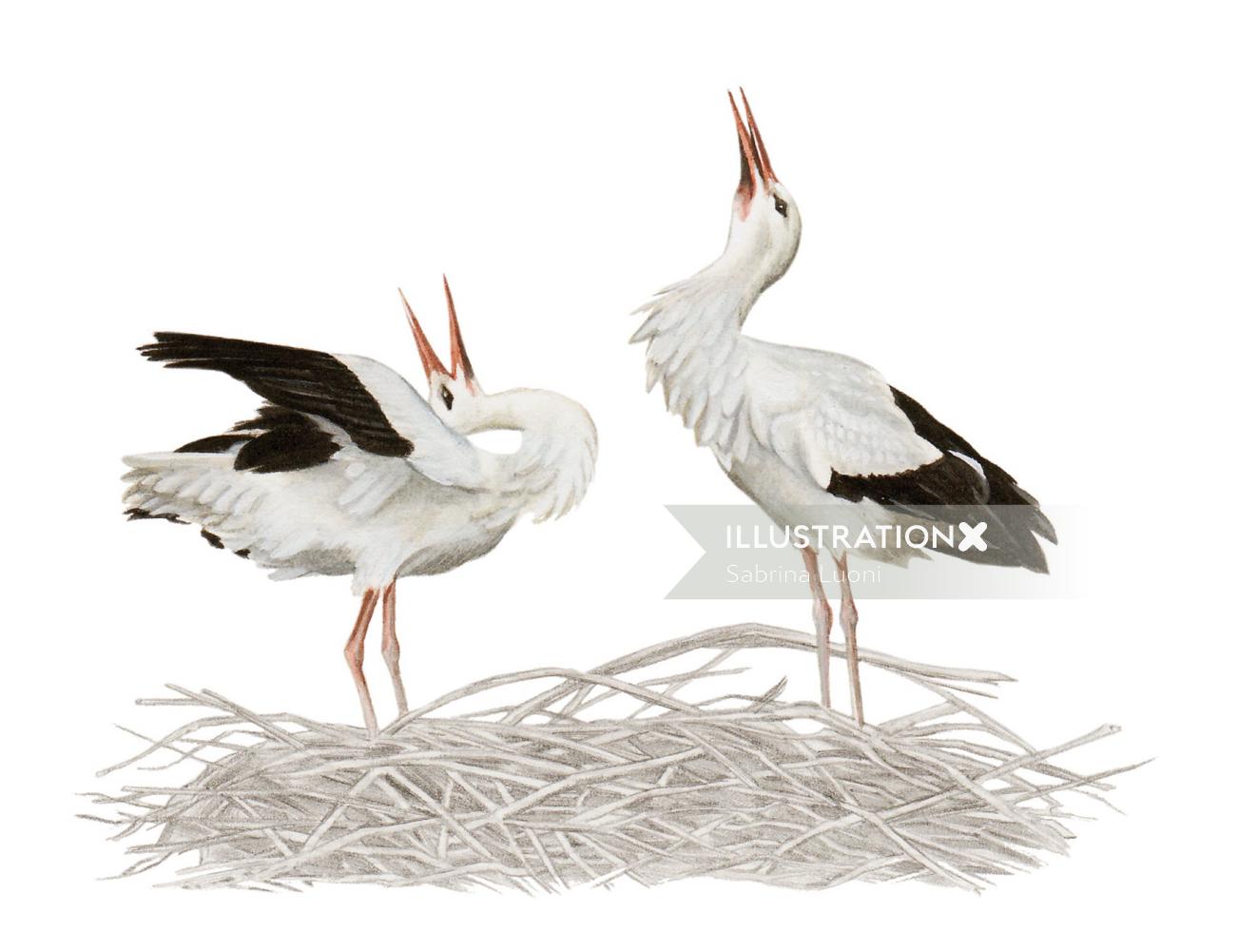This artwork, found on Illustration X and created by Sabrina Luoni, depicts two storks within a nest constructed from a multitude of protruding brown sticks. The storks, with their long, backwards-bending orange legs, are poised with an elegant grace. Each bird is adorned in primarily white feathers, accented with striking black feather tips on their wings. They exhibit long necks akin to swans and sharp, pointed orange beaks. Both storks are depicted with their necks craned upwards, suggesting a sense of alertness or anticipation. The bird on the left appears slightly smaller, with its beak open towards the sky, perhaps awaiting food or communication. This serene and intricate scene captures the delicate beauty of these imposing birds, reflecting a moment of life in their natural habitat.